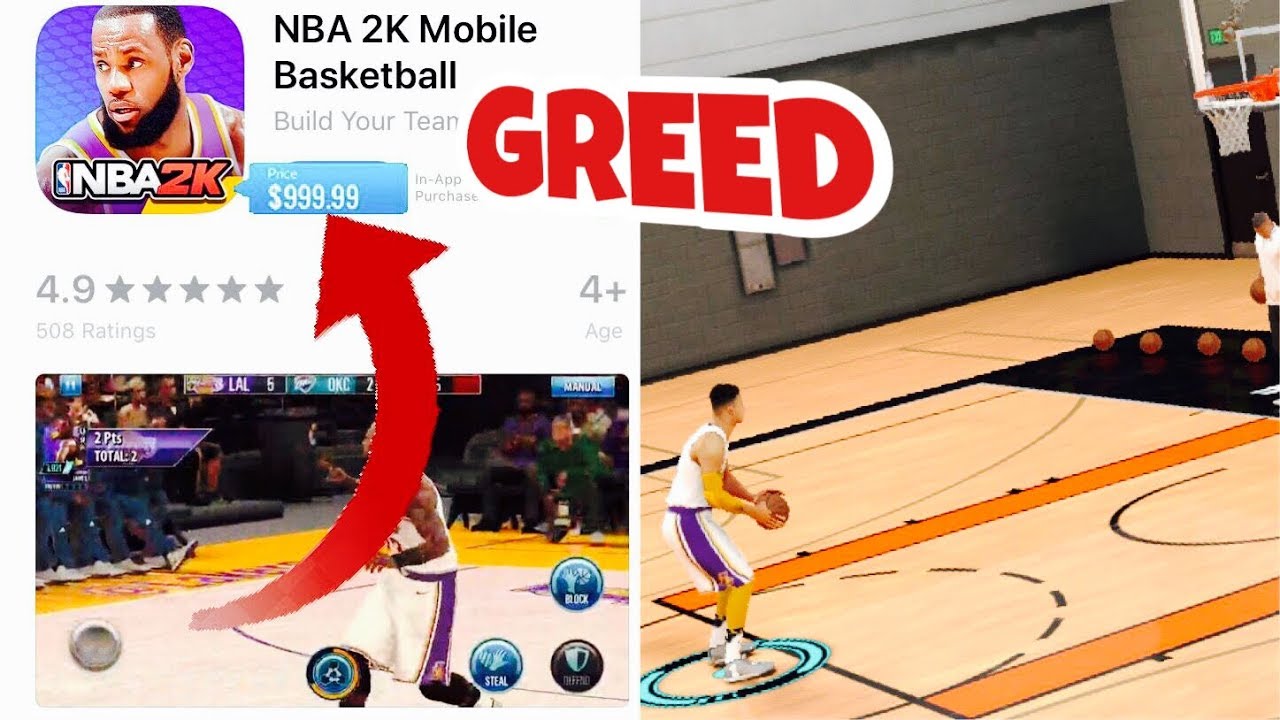The image displays a detailed view of the NBA2K Mobile Basketball app interface, tailored for an iPhone. In the top-left corner, there's the app icon featuring a picture of LeBron James with the NBA2K logo across his chest. Next to it, the app title is clearly printed in bold black text. Below this, the price is prominently highlighted in a blue text box, marked at $9.99. Directly underneath, the app boasts an impressive 4.9-star rating based on 508 reviews, and it is marked as suitable for ages 4 and up.

To the right of the app details, a large screenshot showcases a basketball player at the free-throw line, dressed in a Lakers NBA jersey, exemplifying the game's high-quality graphics. Below that image, another screenshot captures a player on the basketball court, complete with various in-game buttons like "steal," "block," and "defend," and the game score displayed above the player's head.

Dominating the top middle section of the image, bold red text reads "GREED," with an arrow pointing conspicuously at the app's price, insinuating a comment on the app's cost. This detailed composition gives a thorough overview of the app's appearance, functionality, and user reception.